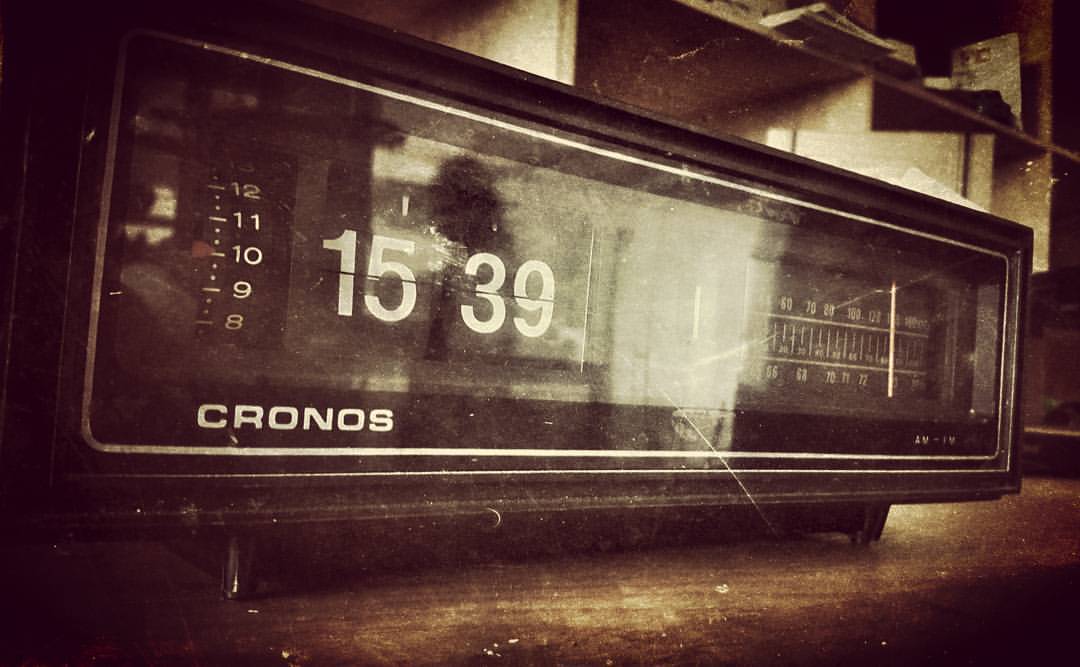A sepia-toned, grainy photograph captures a vintage radio from the 1970s or 1980s. The radio, which rests on a wooden surface, features a digital clock on the left displaying "1539." Adjacent to the clock is a scale ranging from 8 to 12 with a dial set on 10, possibly indicating an alarm function. The bottom of the radio is labeled "Cronos," spelled with a 'C'. On the right side, there is a classic FM/AM radio dial, currently tuned to around 103 FM. The background shows slightly disorganized shelves, adding to the nostalgic atmosphere of the image. The entire scene is rendered in a warm palette of blacks, whites, and browns, emphasizing its retro aesthetic.